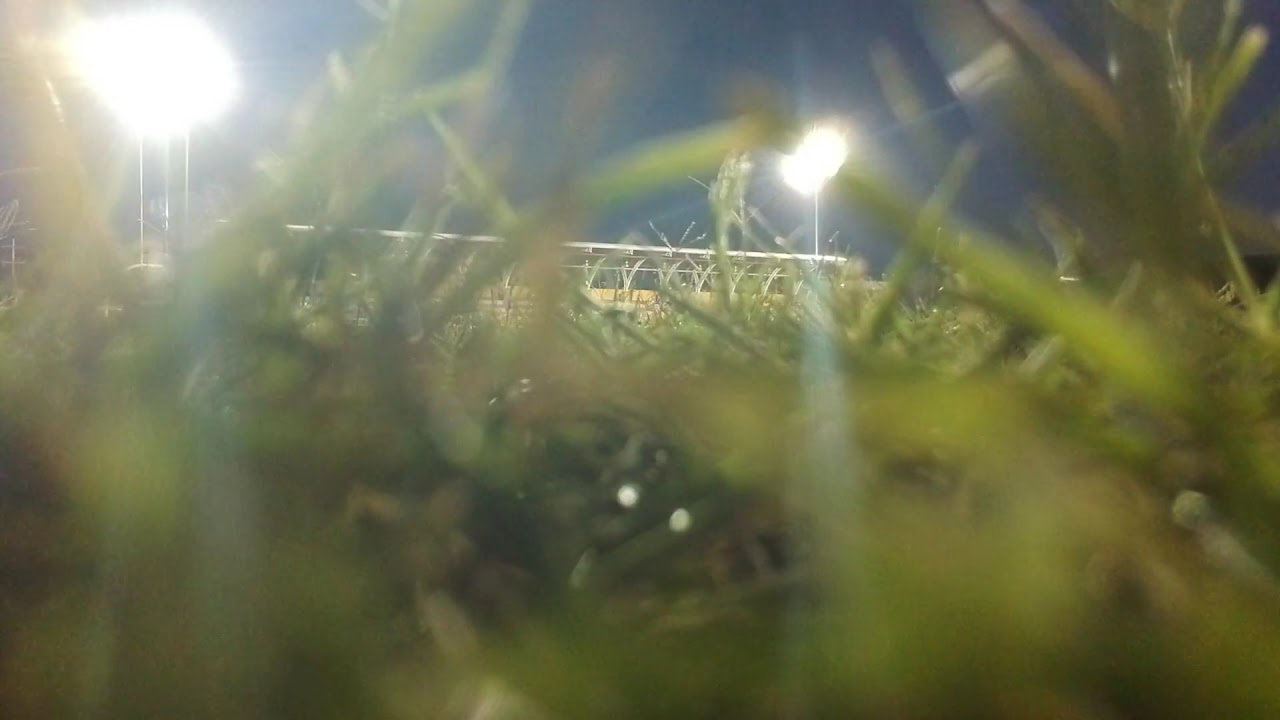The photograph captures an intriguing, almost surreal perspective, reminiscent of an ant’s view of the world. The camera is nestled deep within the grass, looking upward, creating an unusual and immersive viewpoint. The majority of the frame is occupied by blurred blades of grass, their details indistinct, contributing to the sense of proximity and scale. Beyond the grass, the scene reveals an outdoor setting under a dark blue, nighttime sky. Illuminated in the background are bright, almost blinding lights, which could belong to a fence, an elevated roadway, or possibly machinery from a farm. These lights and the silver or gray structure they illuminate lend a sense of industrial or infrastructural presence. The color palette of the image is dominated by greens, yellows, dark blues, and stark whites, merging together in a diffuse, slightly out-of-focus composition that enhances the dreamlike quality of the photograph.